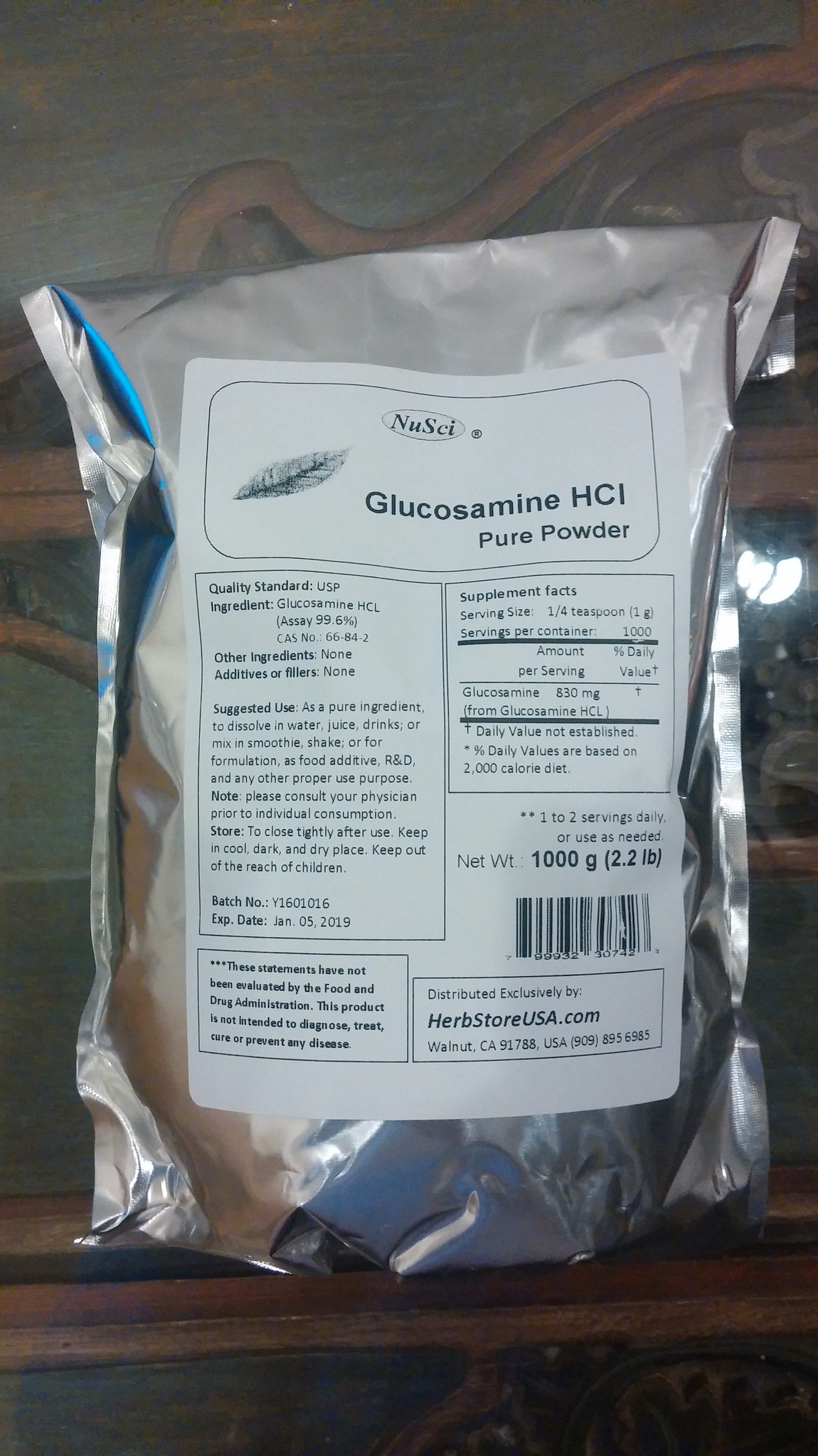In this image, we see a shiny silver package of glucosamine HCl pure powder, standing approximately eight inches high on a dark brown surface. The front of the package features a prominent white label. At the top of the label, the brand name, "NuSci," is printed, accompanied by a grayish leaf graphic. The main text reads "glucosamine HCI pure powder" in black lettering. The package is detailed with various writing on both left and right sides, though much of it is hard to decipher. Additionally, there are several black squares on the label. On the bottom right-hand corner of the label, we can see the website HerbstoreUSA.com, along with the net weight of 1,000 grams (2.2 pounds). Just above the barcode, more detailed product and nutritional information is present but difficult to read due to its small size. The background of the image transitions from lighter to darker shades of green with a hint of a brown frame, emphasizing the package's metallic sheen.